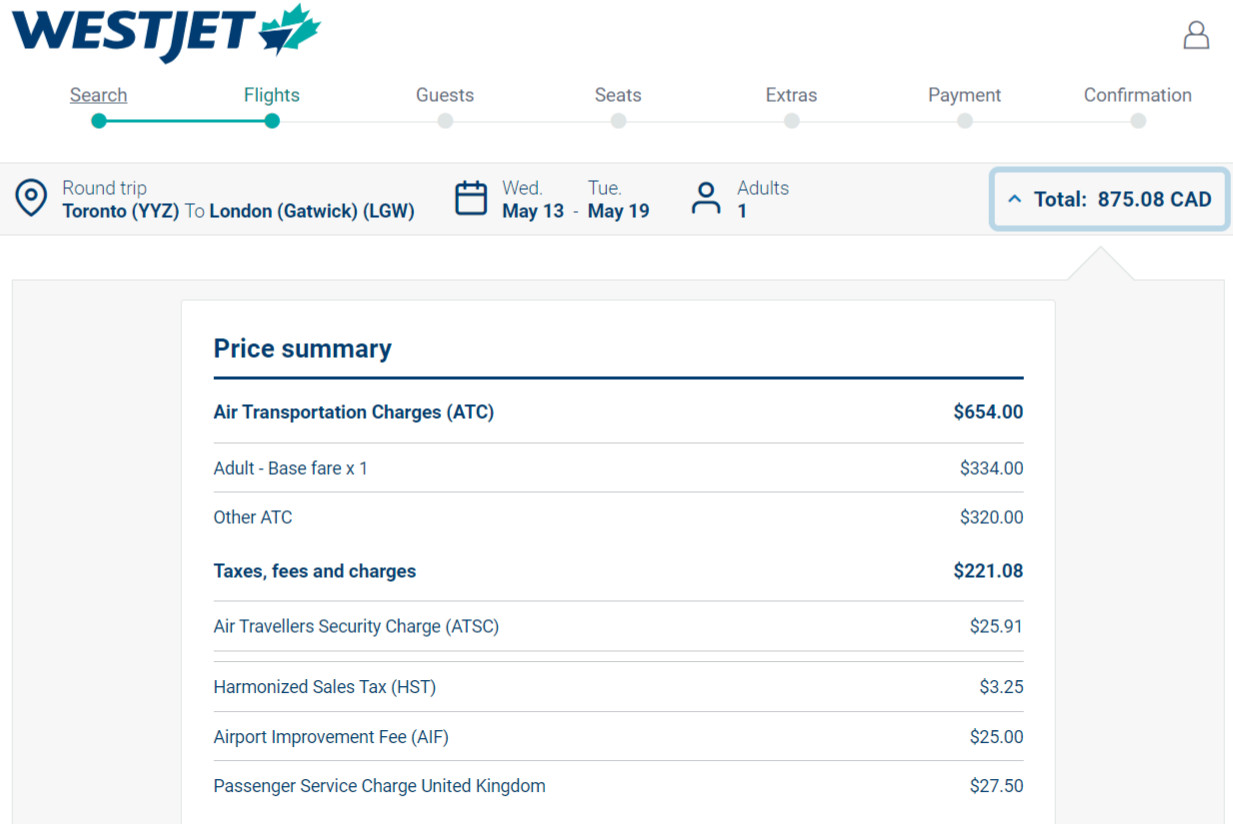**Detailed Caption:**

In this desktop screenshot, the user is navigating the WestJet website, as indicated by the dark blue text and branding. The screen prominently features WestJet's signature blue paper airplane logo flying in front of a stylized maple leaf. Across the top of the interface, there is a progression bar with steps labeled: Search, Flights, Guests, Seats, Extras, Payment, and Confirmation. 

Above the "Confirmation" step, there's a small avatar icon, suggesting that users have the option to sign in.

The currently visible details pertain to a roundtrip flight from Toronto Pearson International Airport (YYZ) to London Gatwick Airport (LGW). The selected travel dates are from Wednesday, May 13th to Tuesday, May 19th, with one adult traveling. The quoted price for this itinerary is 875.08 Canadian dollars.

A detailed price summary breaks down the total cost:
- Airport Transportation Charges (ATC): 654 CAD
  - Adult Base Fare: 334 CAD
  - Other ATC: 320 CAD
- Taxes, Fees, and Charges: 221.08 CAD
  - Air Travelers Security Charge (ATCS): 25.91 CAD
  - Harmonized Sales Tax (HST): 3.25 CAD
  - Airport Improvement Fee (AIF): 25 CAD
  - Passenger Service Charge (United Kingdom): 27.50 CAD

This comprehensive breakdown highlights the various charges and taxes applied to the fare, giving a clear view of the total cost for the roundtrip flight from Toronto to London.